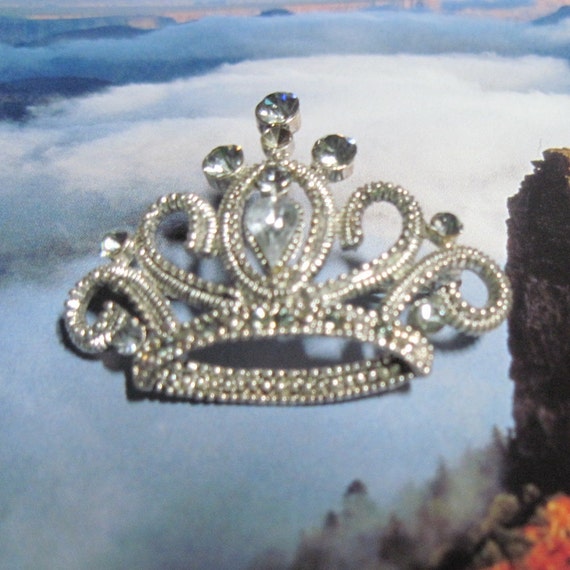The blurry, square photo features a silver tiara adorned with an array of diamond-like jewels, positioned atop a mat that depicts a cloudy sky with a forested landscape in the bottom right corner. The tiara, viewed head-on, showcases a central teardrop-shaped jewel, accentuated by four smaller jewels above it arranged in a pattern with one on each side, two above, and one below. The tiara is uniquely detailed with two rows of gems on each side, curling up and inward toward the central jewel, as well as downwards toward the base. The background, resembling a postcard or page from a book, contrasts the intricate beauty of the tiara with its serene image of a blue sky and clouds, punctuated by a rocky outcrop on the left side.